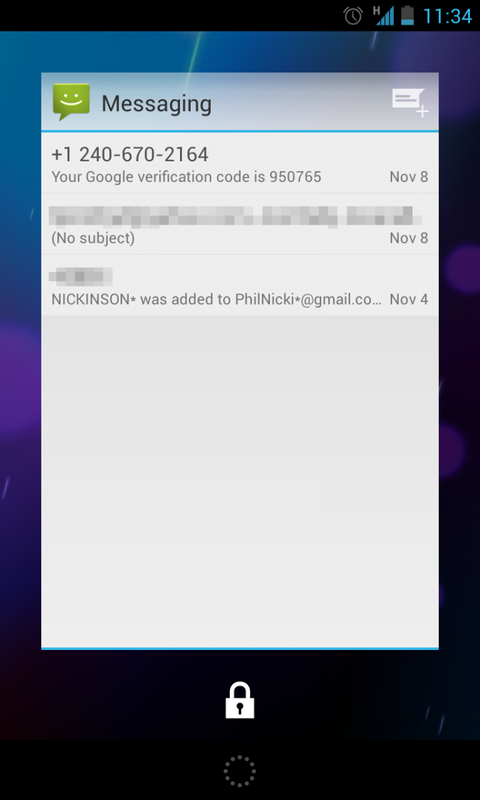This image, captured from a smartphone, showcases the device's wallpaper that features a gradient design. At the bottom, the wallpaper displays black hues transitioning into purple towards the center-left and blue at the top, adorned with purple circles on the right side.

The main focus of the image is an open messaging app. At the top left of the app interface, "Messaging" is displayed in black text on a gray background. Just to its left is a messaging app icon, depicted as a green text box with a smiling throne emoji.

On the upper right corner of the interface, a white conversation box with a plus sign suggests the option to add a new message. Below the "Messaging" header, a blue line separates the top section from the message content.

The displayed messages include:

1. A message from the number +1 (246) 702-164x, dated November 8th, which reads: "Your quickly verified question code is 95075."
2. A second message, partially hidden by a mosaic effect to conceal personal information, labeled "No subject," also dated November 8th.
3. A third message from November 4th, stating: "Nickinson was added to feelunique@gmail.com."

Additionally, a white lock button is visible at the bottom of the interface.